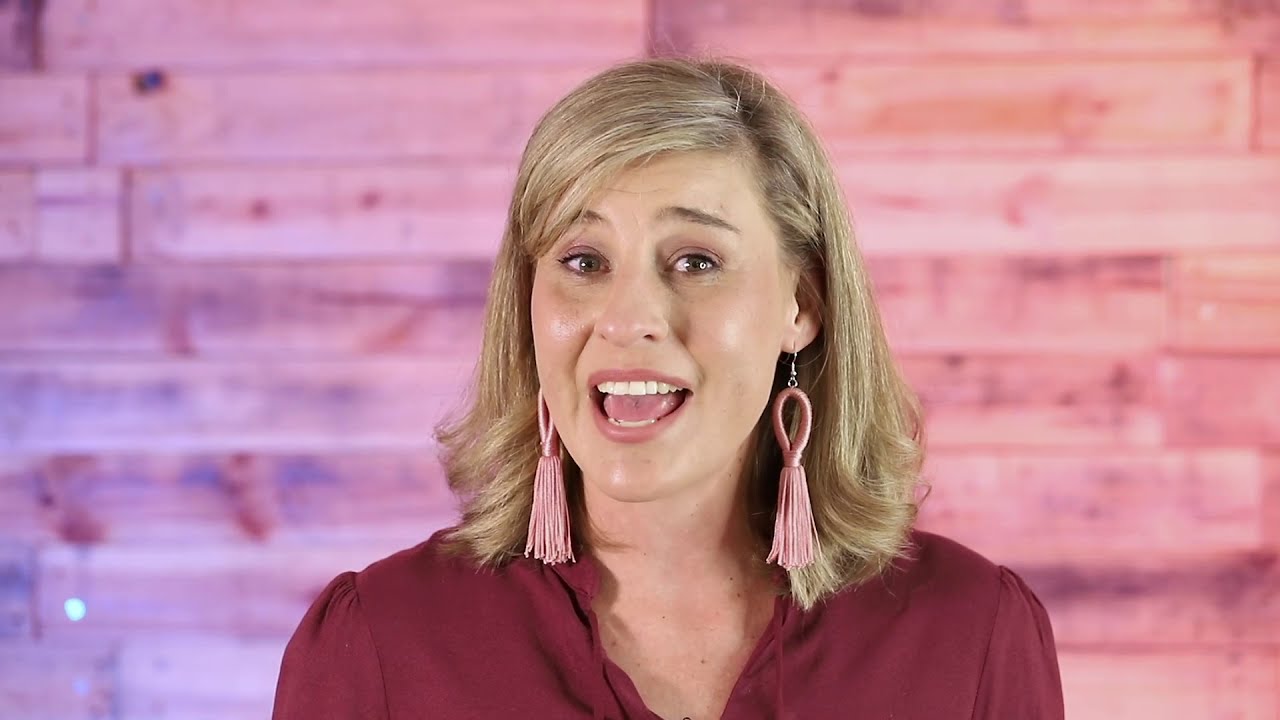The photograph captures a well-lit image of a woman with shoulder-length, blonde or very light brown hair, parted on the side, wearing a red button-down shirt. She's in mid-sentence, her mouth open, and eyebrows slightly raised, conveying an expression of interest and passion in what she's discussing. She has dangly, pink hoop earrings adorned with tassels. The background is slightly blurry, composed of wooden panels reminiscent of a cabin's interior, featuring reddish-orange and brown tones. The camera is positioned at the height of her head, approximately three feet away, framing her from the chest up and focusing sharply on her face as she gazes directly into the lens with her head slightly tilted to the right.